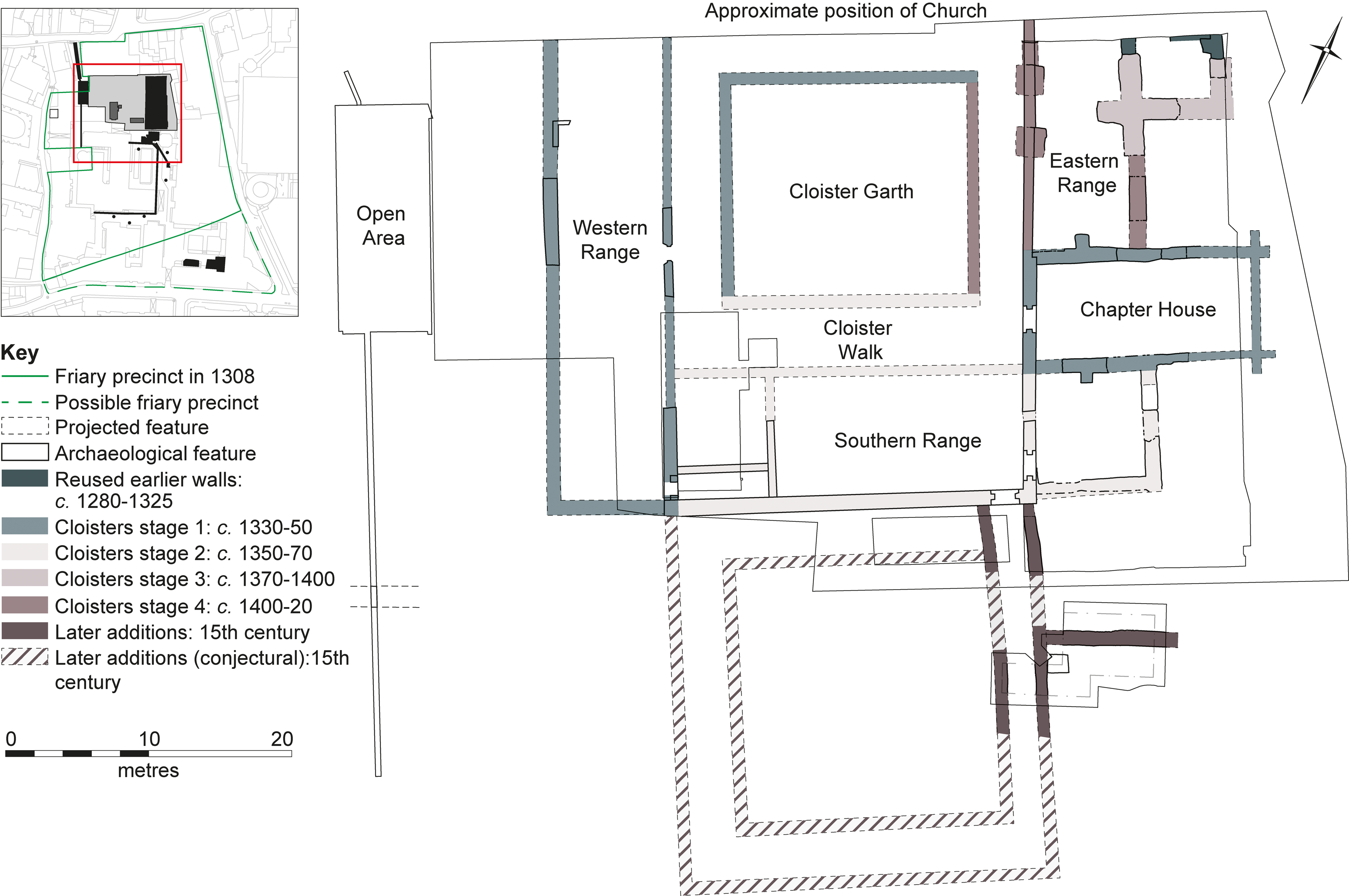The image depicts a detailed blueprint of a church and its surrounding buildings. At the top of the diagram, it is labeled "approximate position of church" in black text. The central area, marked as "Cloister Garth," is bordered by significant architectural elements. To the left of Cloister Garth is the Western Range, and to the right is the Eastern Range. Directly below the Cloister Garth runs the Cloister Walk, beneath which lies the Southern Range. Adjacent to the Eastern Range and below the Cloister Walk is the long rectangular Chapter House. 

The bottom section of the blueprint displays dashed squares, with one contained within another, though they are unlabeled. On the left side of the image, a zoomed-out portion shows the church's placement within a possible cityscape, with a red square highlighting the specific building detailed in the blow-up to the right. Below this, a key identifies various elements of the map, including a green line labeled "Friary Precinct in 1308" and a dashed green line denoting a "possible Friary Precinct," alongside other cloisters and structures. The map uses a color-coded scheme with a range of colors from dark blue to brown and gray to outline different areas and features of the church, indicating a comprehensive and detailed architectural layout.